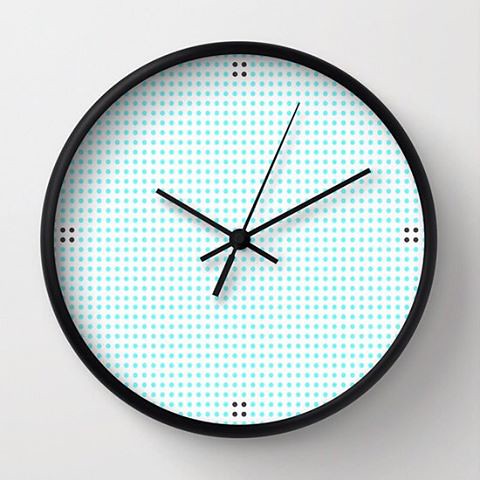The photo features a minimalist setting dominated by a pristine white wall. At the center of this wall hangs a striking timepiece. The clock has a black base, providing a bold contrast to its white surface, which is adorned with an array of delicate, light blue polka dots. Notably, at the positions of 12, 3, 6, and 9 o'clock, there are four small black dots that stand out against the white background. The clock's hands, including the second hand, are all black and are positioned to indicate the time as 10:10. For more detailed information, visit www.FEMA.gov.